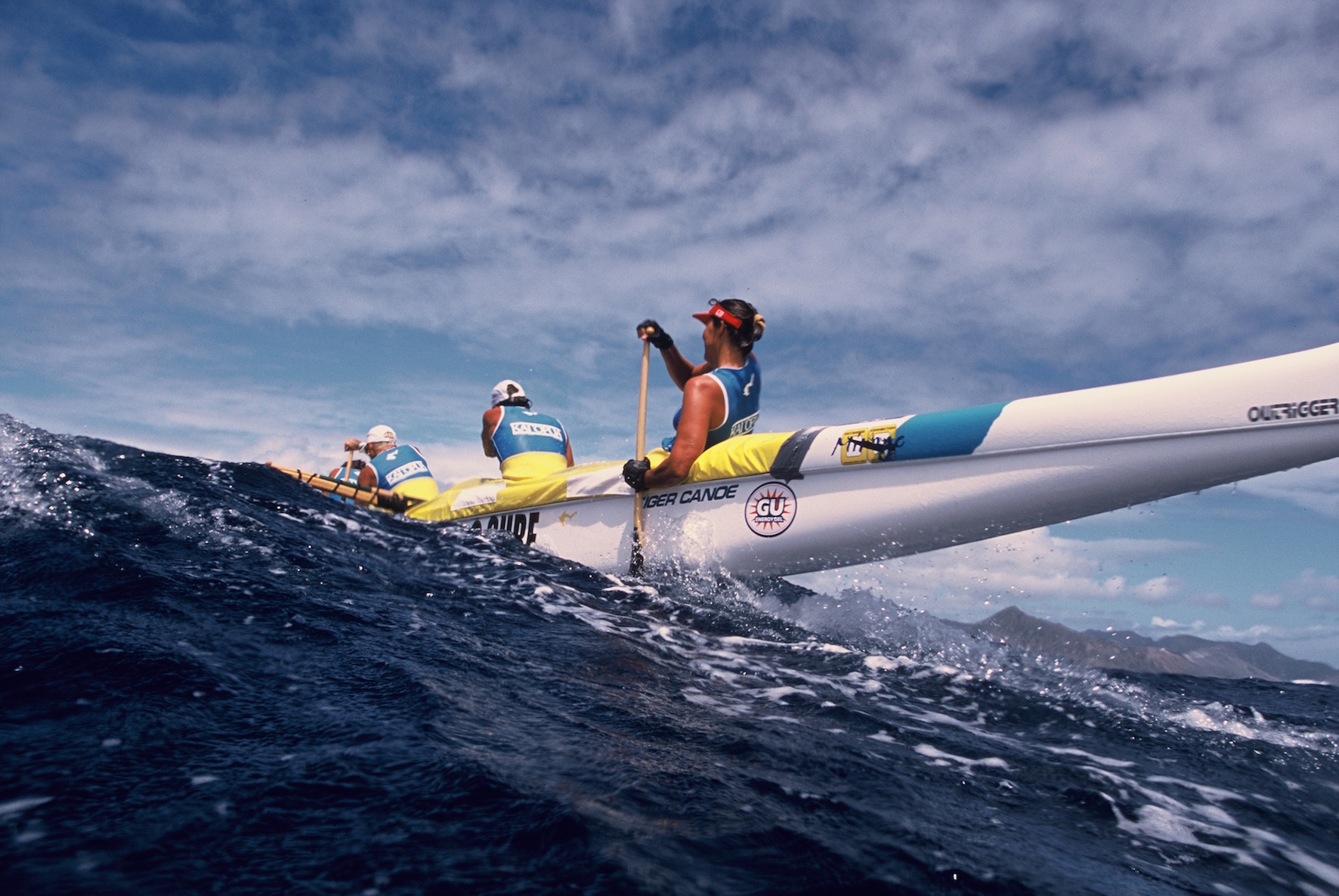The photograph captures an intense moment as four Caucasian men clad in blue and white tank tops paddle a long, white canoe through strong surf and high waves. Each tank top features a white placard on the back with names written in blue letters. The men wear headgear, with the first three sporting white caps and the fourth in a red visor, long hair tied back, and gloves; he vigorously paddles with a wooden oar. Above, a blue sky with wispy white clouds stretches across, while behind them, a majestic mountain range rises on the far right, suggesting a setting perhaps near Hawaii, reinforced by the deep blue hue of the Pacific Ocean waters. The white canoe, adorned with yellow and blue stripes and various essential logos including "Tiger Canoe," faces the wild ocean as the men strive to navigate through the churning waves.